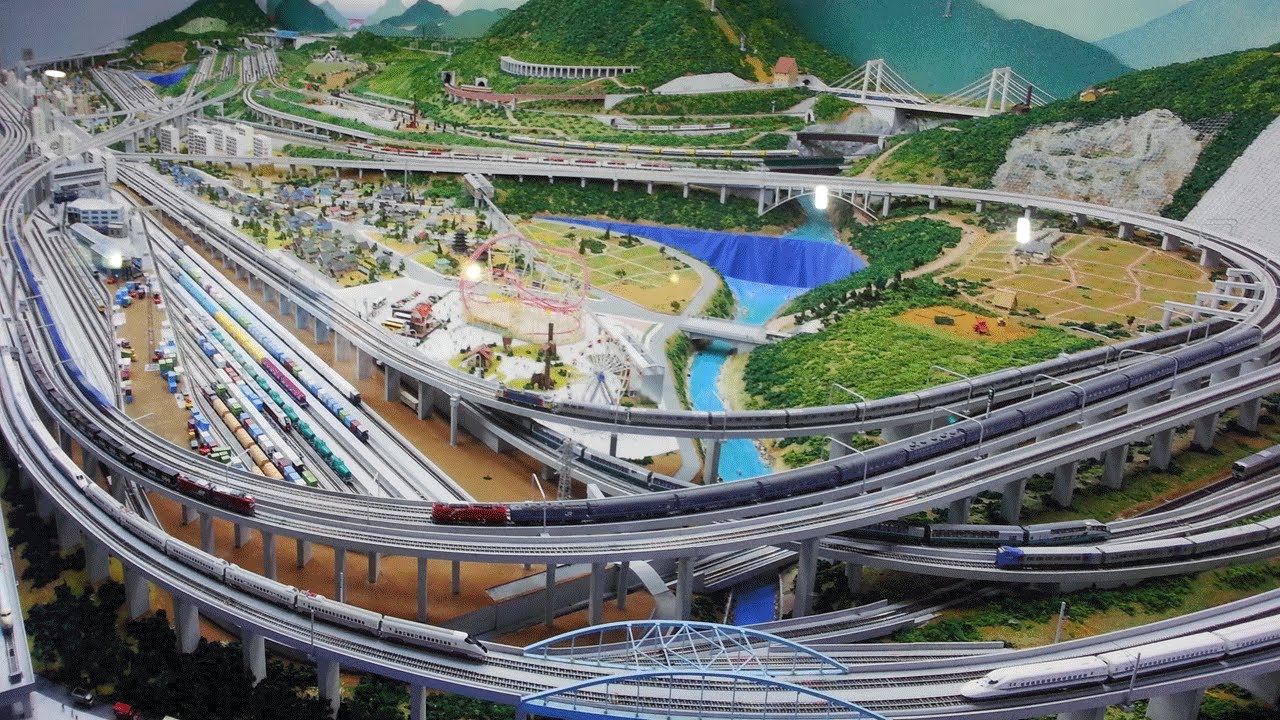The photograph depicts a detailed model train set of a futuristic city. The train tracks form an oval looping continuously from left to right, with the left side densely packed with tracks and what appears to be a station. The model showcases about three loops of tracks, with protruding railways at the top and bottom. Stationary trains are seen towards the bottom, represented in shades of gray and white, evoking a modern design. Surrounding the central train tracks is a diverse landscape featuring a river with a bridge, various pathways resembling roads, and expanses of light and dark green terrain.

To the left, there are parked trains in vibrant colors such as yellow, red, and green. Dominating the scene at the top center is a large white bridge beside a significant mountain or hillside, colored in verdant hues. The depiction includes numerous roads and highways, accentuating the city's intricate transportation network. Additionally, a substantial blue river, green mountains, and cylindrical structures suggestive of either roads or racetracks contribute to the dynamic and futuristic character of the model cityscape.